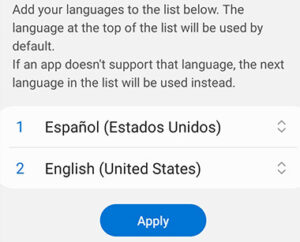This is a screenshot from an unidentified webpage featuring a gray background. At the top of the screen, an instructional message reads, "Add your languages to the list below. The language at the top of the list will be used by default. If an app doesn't support that language, the next language in the list will be used instead." Below this message are two white rectangles arranged in a vertical list. The first rectangle, marked with a blue number "1," displays the text "Español (Estados Unidos)." The second rectangle, marked with a blue number "2," shows "English (United States)." At the bottom of the screen is a dark blue oblong button with the word "Apply" centered in white lettering. The screenshot does not contain any illustrative or photographic elements, and there are no visible people, animals, birds, plants, flowers, trees, buildings, bridges, flags, banners, signs, billboards, automobiles, helicopters, or airplanes.